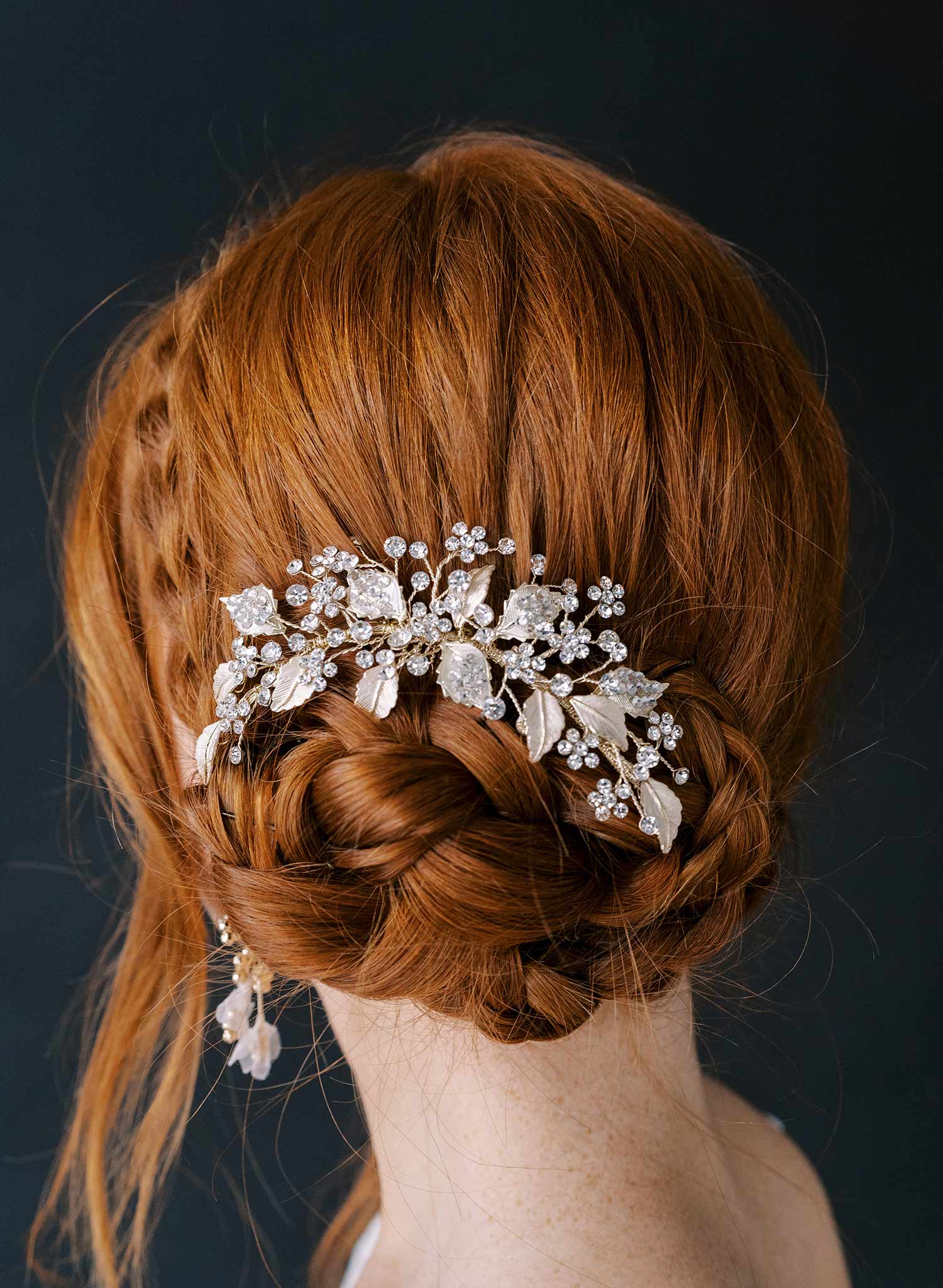This color photograph features a woman of European descent with strikingly vivid reddish-ginger hair styled in an elegant updo. The background is a dark grayish-black hue, accentuating the rich color of her hair and the intricate details of her hairstyle. Her hair includes a French braid originating from the top of her head, flowing seamlessly into an intricate bun made up of twisted and wrapped braids. A delicate wisp of hair escapes from the bun on the left side, adding a touch of natural elegance.

The updo is adorned with a sophisticated hairpin shaped like a silver leaf, encrusted with white or clear crystal rhinestones arranged in small branches or flowers. This ornate pin, also referred to as a hair comb, complements her matching dangling earrings, which carry a harmonious design theme with diamond-like studs and possibly gold accents. The combination of her elaborate hairstyle and the luxurious accessories creates a captivating and refined look.